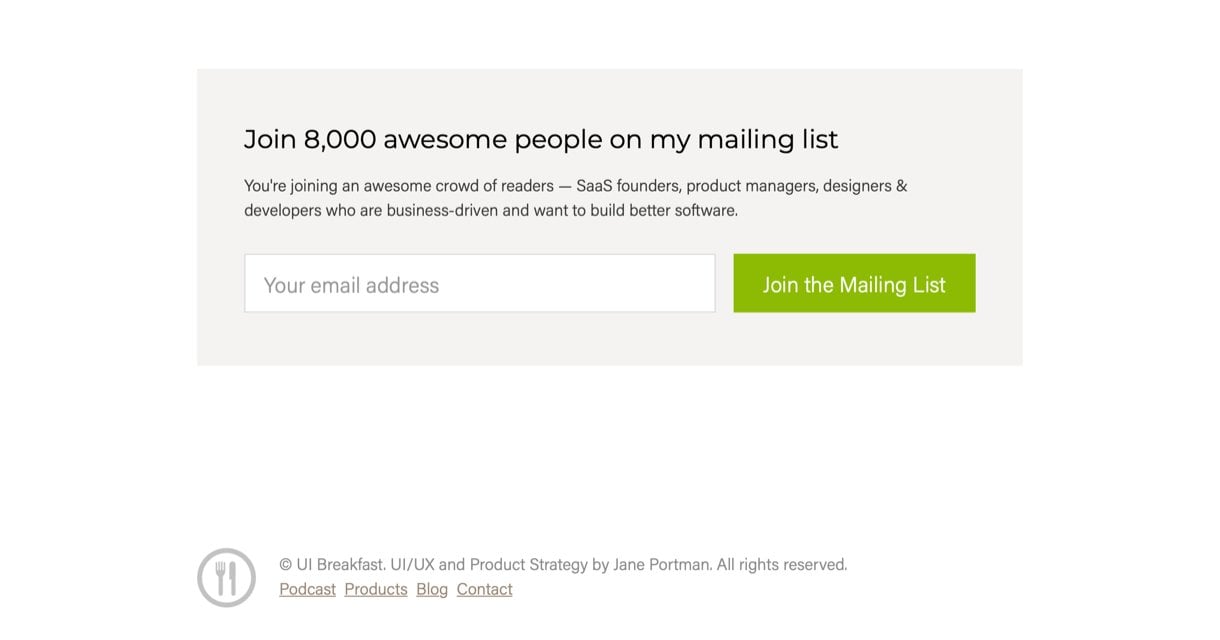This image depicts the lower section of a web page with a clean, white background. A light gray pop-up window is featured prominently at the top section of this area. Inside the pop-up, there's a call-to-action inviting users to join a mailing list. The text reads: "Join 8,000 awesome people on my mailing list. You’re joining an awesome crowd of readers - SaaS founders, product managers, designers, and developers who are business-driven and want to build better software." Below this text, there's an input field prompting users to enter their email address. Adjacent to this field is a green button labeled "Join the Mailing List."

At the very bottom of the page is a circular icon containing a fork and knife symbol in gray. To the right of this icon, the text "UI Breakfast - UI/UX and Product Strategy by Jane Portman. All rights reserved" is displayed. Directly following this is a navigation menu listing options such as "Podcast," "Products," "Blog," and "Contact."